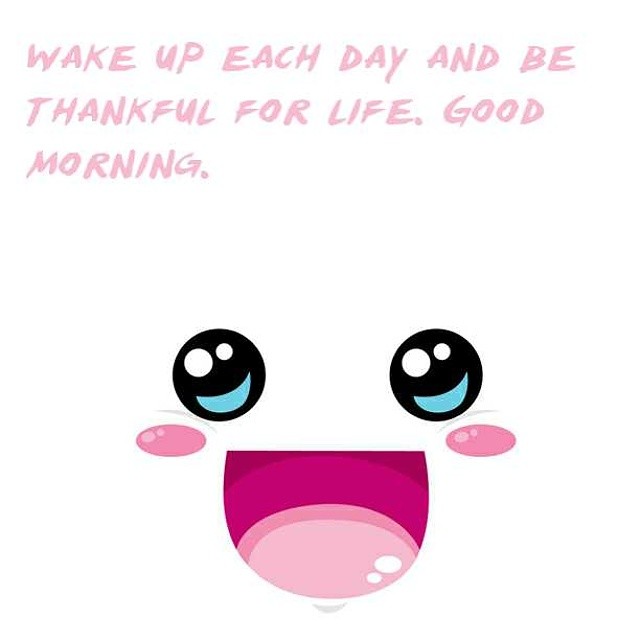The image features a bright white background with light pink text at the top, written in uppercase letters that read, "Wake up each day and be thankful for life. Good morning." Below the text is an anime-inspired cartoon face. The face consists of large, circular black eyes with blue semi-circles and white reflections, giving them a sparkling appearance. It has two round, egg-shaped pink cheeks with a slight sparkle. The mouth is a large, half-circle shape resembling a cup, with varying shades of pink, and a visible pink tongue. This detailed illustration captures a cheerful and uplifting emotion.